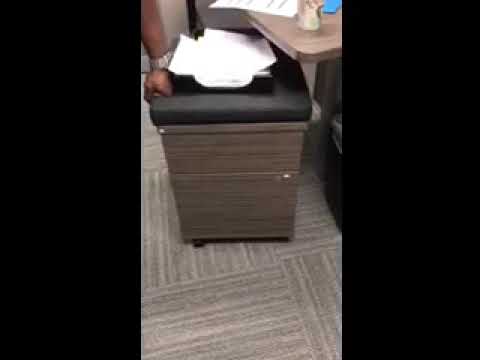The image captures an indoor setting with a central piece of furniture that appears to be a gray bench featuring drawers, topped with a padded surface. This piece resembles a nightstand due to its drawer design but is likely meant to function as a seating area, suggested by its padded top. A man's hands are interacting with the furniture; one hand attempts to pull open a drawer, while the other rests on the padded top. The individual wears a silver wristwatch on his left wrist, though his full body is not visible in the frame.

The bench is positioned centrally on a gray-tiled carpeted floor. On the padded top lies a white piece of paper. Adjacent to the bench is a gray and beige table, which holds a coffee cup, a blue envelope, and a partly visible piece of paper with illegible text. The room is brightly lit, suggesting it's captured in daylight. In the background, additional elements such as the brown table suggest an office-like environment. The image seemingly forms the central panel of a triptych, flanked by black panels on each side.